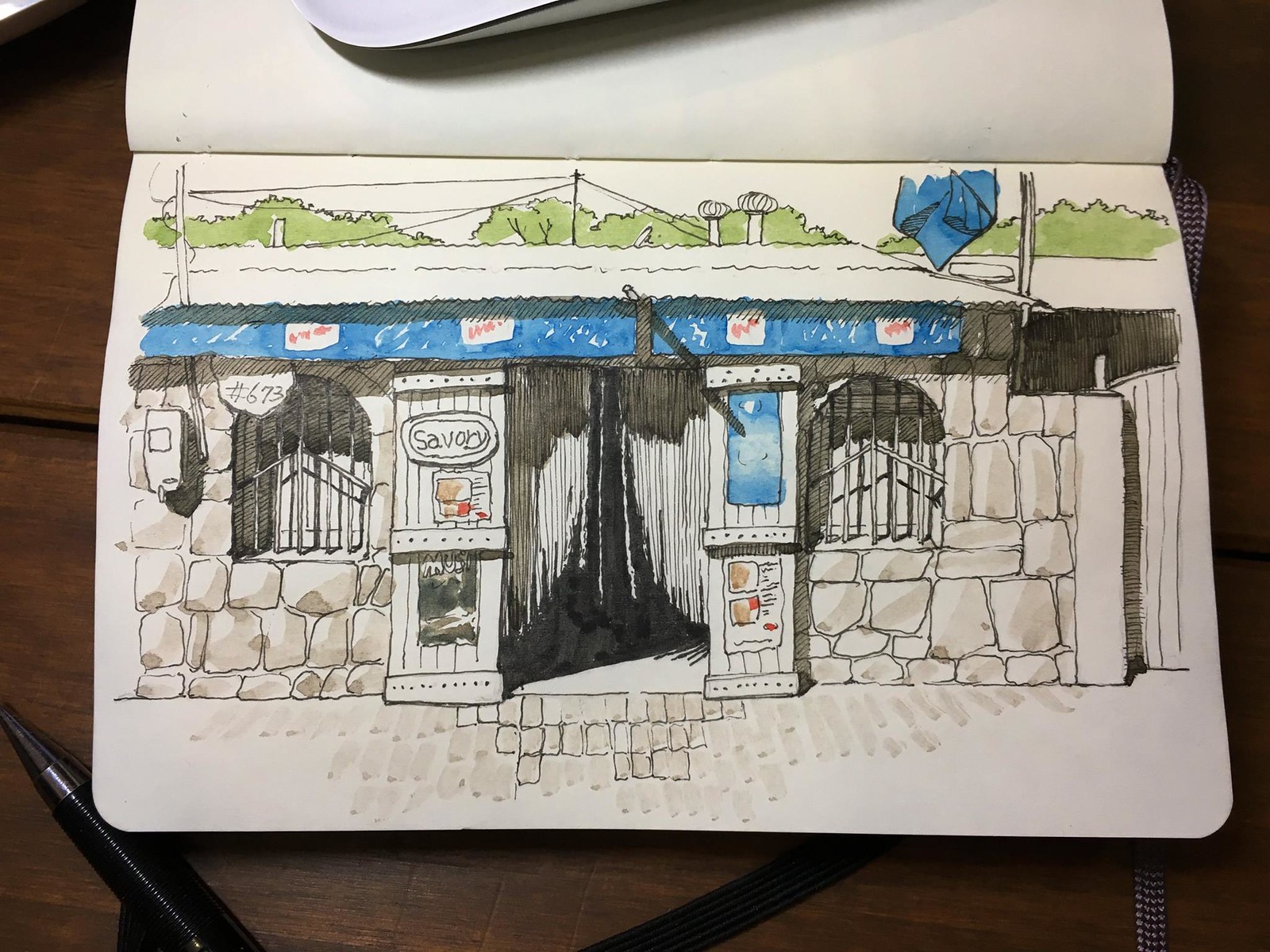The image features a close-up of an intricately drawn illustration of what appears to be a quaint tavern or bar. The structure of the tavern is rendered in fine white lines, set against a richly textured background composed of numerous stones and slabs of marble. The front door, partially veiled by white tassels, stands slightly ajar, inviting curious onlookers to imagine stepping inside. 

Although the interior details are obscured, subtle hints suggest the presence of small animals, possibly a tiny white dog, nestled in the backdrop of the establishment. The signage prominently displays the word "Savory" as the tavern's name. Just below, the number 673 is clearly visible, marking the address. Above the sign, a blue shingle is adorned with four small, red and white pieces of paper, though their specifics remain indistinct. The scene is further enriched by the delicate addition of green trees visible in the distance, blending the tavern into a serene and picturesque environment.